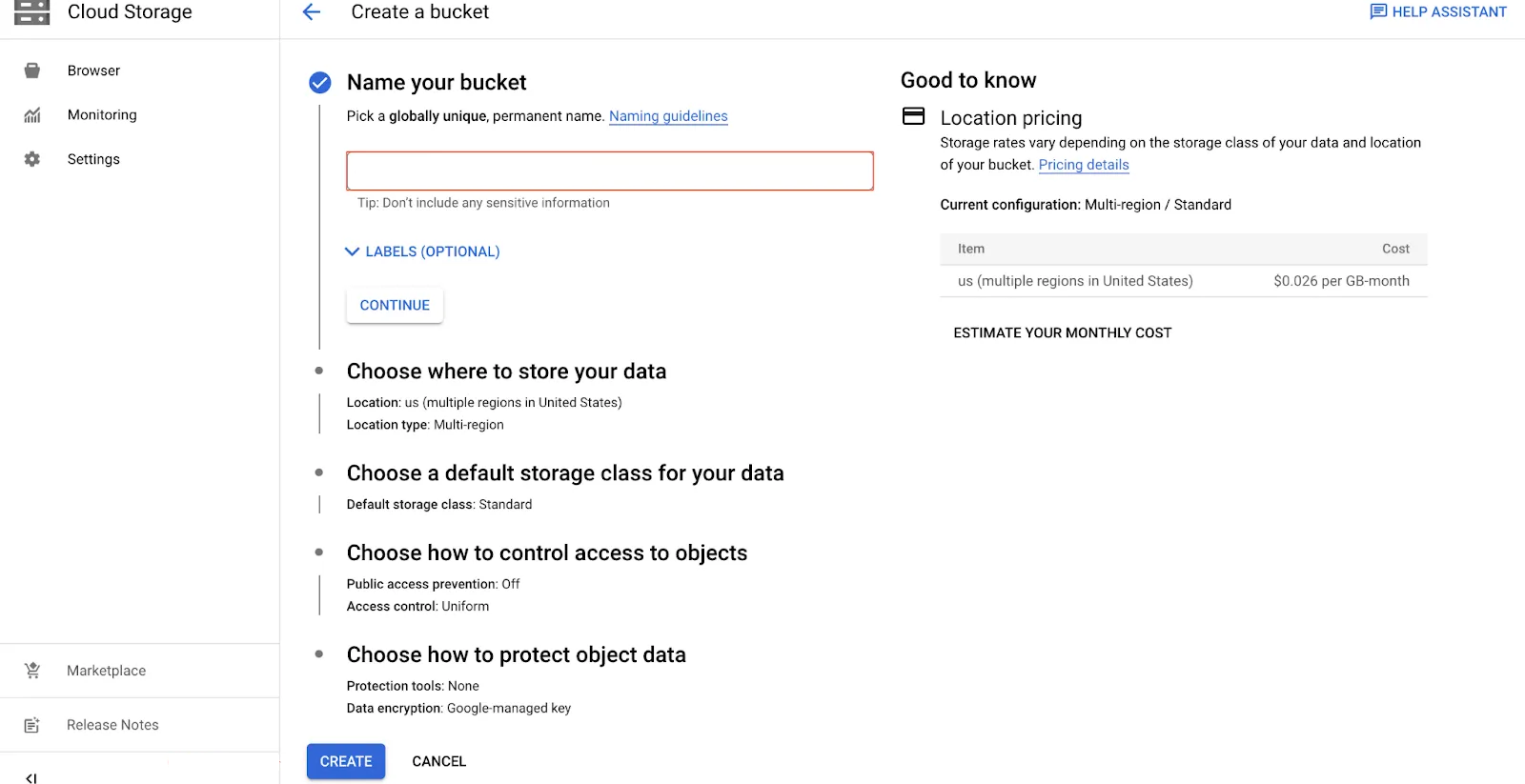The image is a horizontally rectangular screenshot from a Cloud Storage interface with a clean, white background. In the upper left corner, the title 'Cloud Storage' is prominently displayed. To its right on the same line, there is a blue back arrow icon followed by the option to 'Create a bucket.' Further to the right, the word 'Help' is shown in blue text.

On the left side of the interface, there is a vertically oriented column of navigation options including 'Browser,' 'Monitoring,' and 'Settings.' Near the bottom of this column, 'Marketplace' and 'Release Notes' are listed.

Beneath the 'Create a bucket' option, several headings outline the steps and settings for bucket creation. These include:
1. Name your bucket - accompanied by a field to enter the bucket name.
2. Choose where to store your data.
3. Choose a default storage class for your data.
4. Choose how to control access to objects.
5. Choose how to protect object data.

Below these options, a blue 'Create' button is visible, with a 'Cancel' button beside it.

To the right of the step-by-step process, there is an informational section titled 'Good to know.' This section includes details on location and pricing:
- Storage rates vary depending on the storage class of your data and the location of your bucket.
- Current configuration: Multi-region, standard item.
- Location: US, multiple regions in the United States.
- Cost: $0.026 per gigabyte-month.